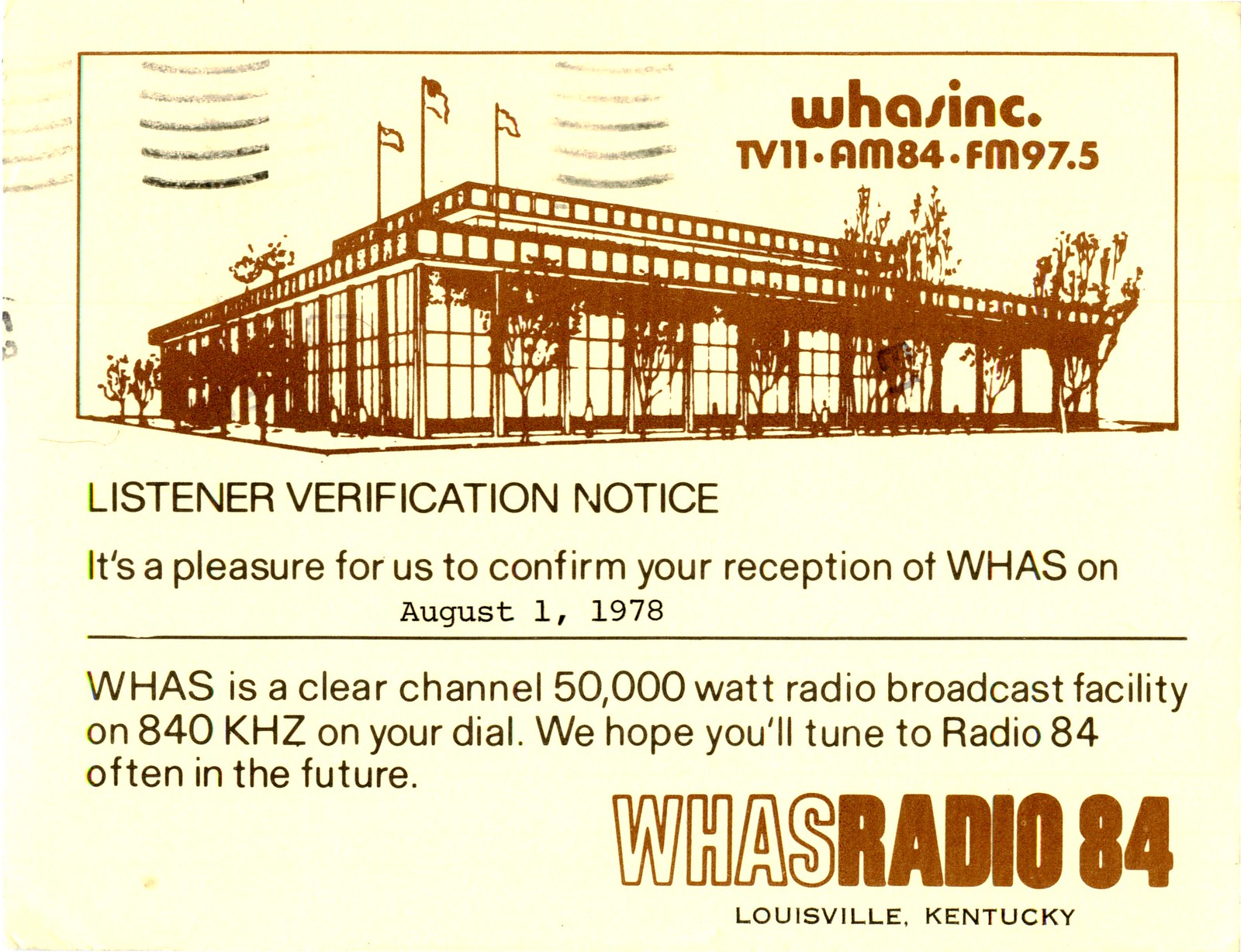The image appears to be a stylized postcard featuring a detailed illustration of a large, rectangular building with extensive glass sides, surrounded by trees. The building has three flagpoles located toward the center left. The background of the postcard is cream-colored, while the text ranges from brown to black, with the prominent brown illustration of the building dominating the upper section. At the very top right, it reads "WHAS INC TV 11 AM 84 FM 97.5" in brown text. Across the top left and center, horizontal wavy lines suggest postal markings. Below the building illustration, the text announces: "Listener Verification Notice: It's a pleasure for us to confirm your reception of WHAS on August 1st, 1978." A horizontal line separates this section from additional information, which states: "WHAS is a clear channel 50,000-watt radio broadcast facility on 840 KHz on your dial. We hope you'll tune to Radio 84 often in the future." At the bottom right, the WHAS logo appears; it's presented in cream color with a brown border and reads "WHAS Radio 84" in full brown text, followed by "Louisville, Kentucky" in smaller black letters.